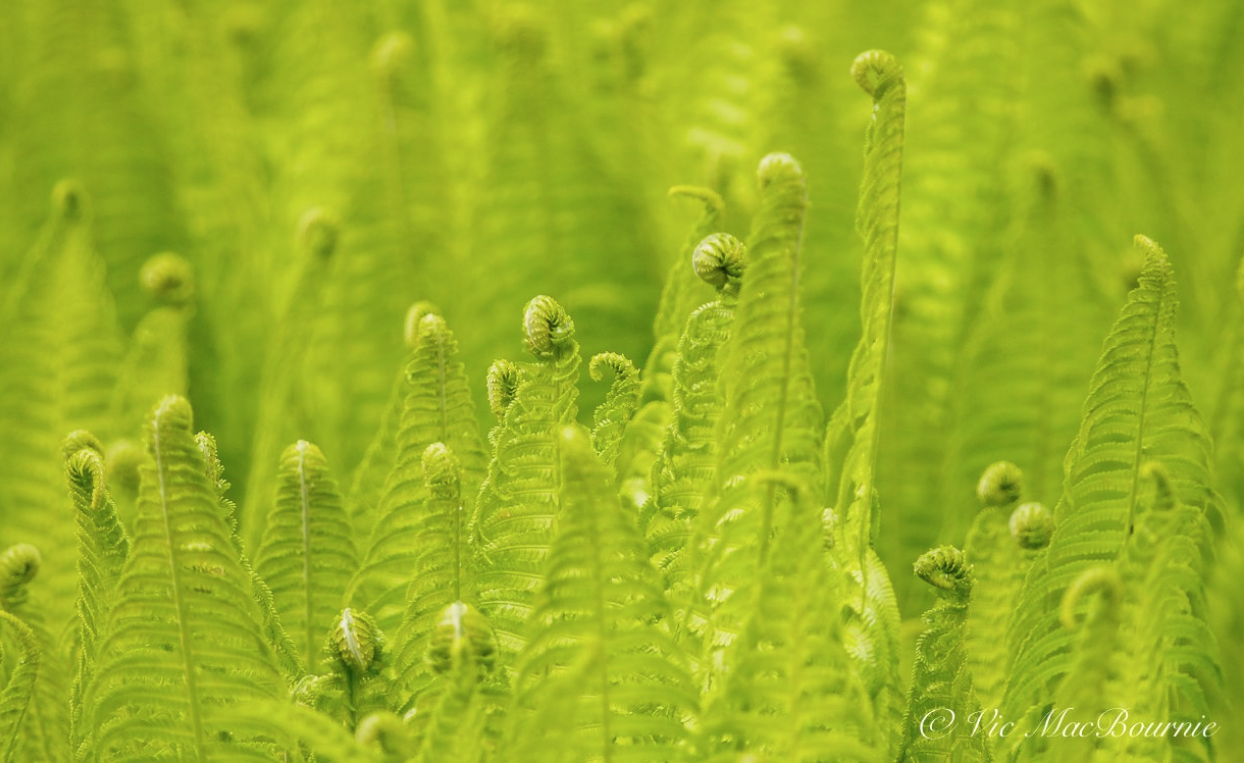A verdant scene featuring a close-up of plants with a verdant hue dominates the picture. The vertical plants have triangular-shaped leaves with a central stem adorned with horizontal lines radiating outward. The top of each plant thins and curls gracefully, with some stems showing a hint of white where they bend. The leaves display gentle curves along their margins. The background is blurred, showcasing more of the same lush greenery, enhancing the focus on the foreground plants. In the bottom right-hand corner, the name "Vic McBurney" is elegantly inscribed in cursive white font, adding a personal touch to the vivid green composition.